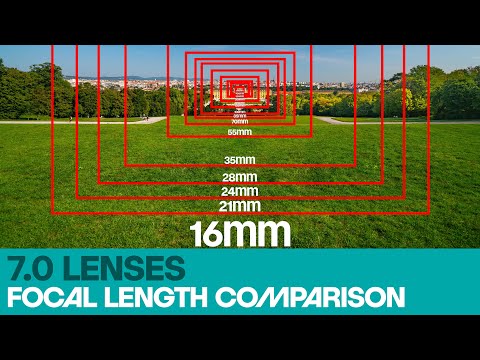The image is a detailed focal length diagram set against a vibrant park scene within an urban environment. The park itself is an expansive, well-maintained grassy lawn encircled by lush trees, with a clear blue sky and cityscape visible on the horizon. Superimposed on this picturesque background are multiple concentric red rectangles, each labeled with a corresponding focal length: 16mm, 21mm, 24mm, 28mm, 35mm, 55mm, 70mm, and continuing into the distance. These rectangles demonstrate the varying field of view captured by different lenses. Centered at the bottom of the image is a turquoise bar inscribed with "7.0 Lenses" in dark blue text, and just below it, in bold white letters, the phrase "Focal Length Comparison" is prominently displayed. Additionally, faint silhouettes of people walking along a concrete path provide a sense of scale and activity within the park.